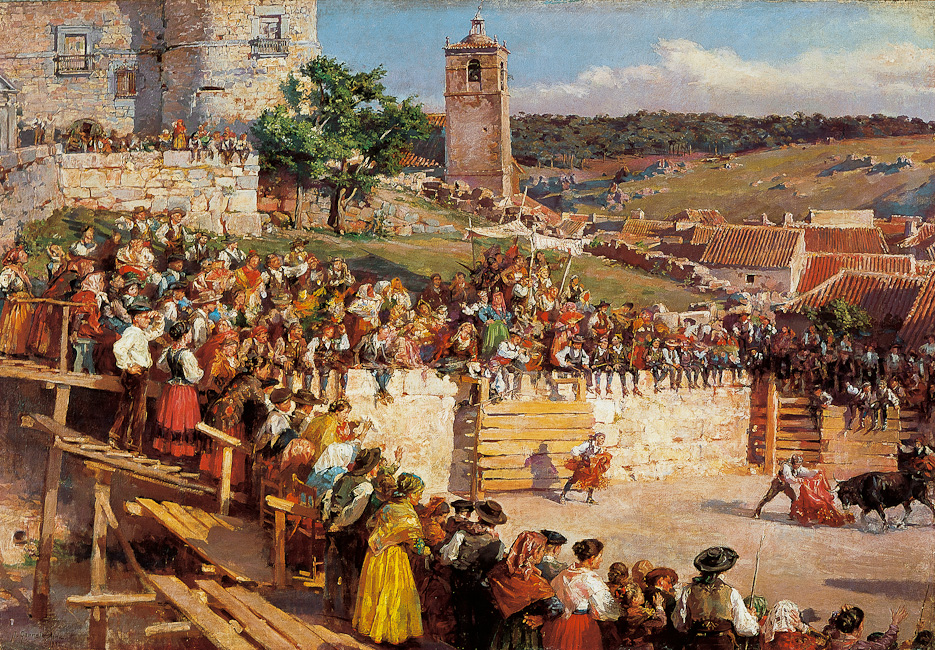This vivid and detailed oil painting depicts a lively 19th-century Spanish bullfight in a vibrant outdoor scene. Dominating the central distance of the composition, a tall guard tower, reminiscent of the 17th century, rises against a blue sky peppered with gray clouds. Located towards the top left, a stone building crafted from yellow stone adds historical depth to the setting. The background showcases green hills adorned with trees and shrubs, along with traditional terracotta-roofed homes that echo the Spanish landscape.

A significant portion of the painting features a bustling crowd in colorful, traditional Spanish attire from the 1800s, engaging with the spectacle below. The women are adorned in long dresses with capes or scarves draped across their shoulders, some with scarves on their heads, while the men sport vests or white shirts. They gather around a wooden-railed raised platform, their attention intensely focused on the courtyard below, where the central bullfighting action unfolds.

In the foreground, two bullfighters wielding red capes confront a charging bull. The bull is depicted mid-charge, aiming towards the bullfighter on the right, who holds his cape outwards to capture the bull’s attention. The other bullfighter keeps his red cape close to his chest, positioned a few feet behind. Nearby, young boys sit precariously on a fence close to the edge of the bull pit, adding a sense of youthful daring and anticipation to the scene. The stone enclosures and wooden structures serve as viewing platforms, ensuring the safety of the onlookers while providing them with an unobstructed view of the thrilling tableau below.